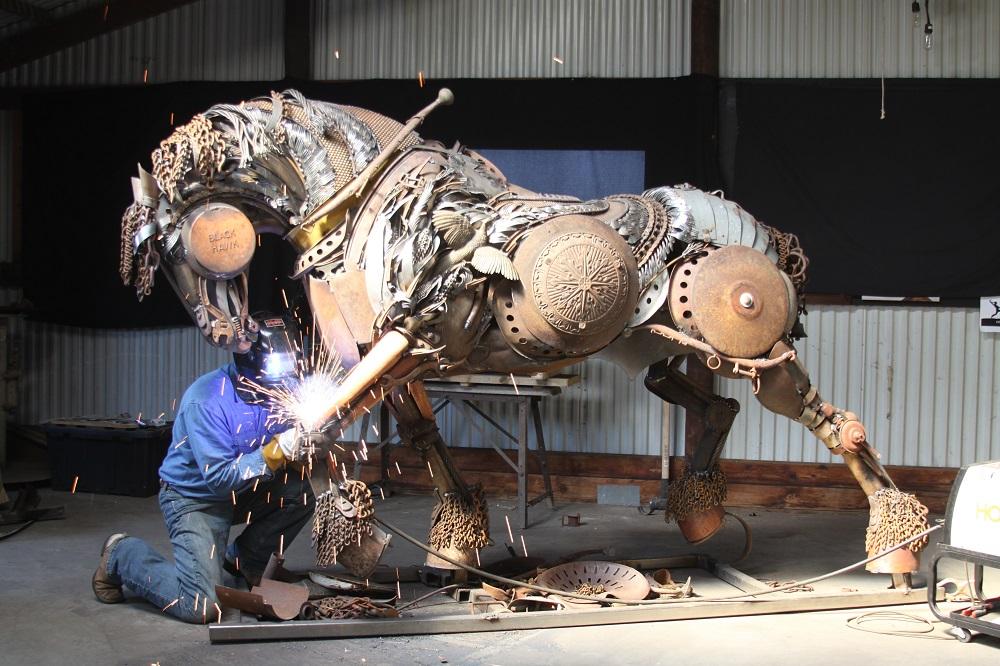In the center of the image, a man is captured in the act of welding a large, intricately crafted metallic sculpture of a horse. The statue, resembling the height of a man, is composed of various recycled metal pieces, providing a detailed, textured form. The horse's mane is formed from chains, while its cheek is ingeniously crafted from a cast iron pan. The midsection features a shield, and above the hooves, more chains are evident. The limbs are constructed from rivets and steel bars, and the rear end incorporates a piece of shoulder plate armor, completing its armored appearance. Below the horse's head, the man kneels, focused on welding the front leg. Sparks fly from the welding torch he holds. He is equipped with a black welding helmet, a blue long-sleeved shirt, blue jeans, heavy yellow gloves, and brown boots. Behind this intricate scene, the white, riveted shed wall sets a contrasting background, highlighting the creative endeavor.